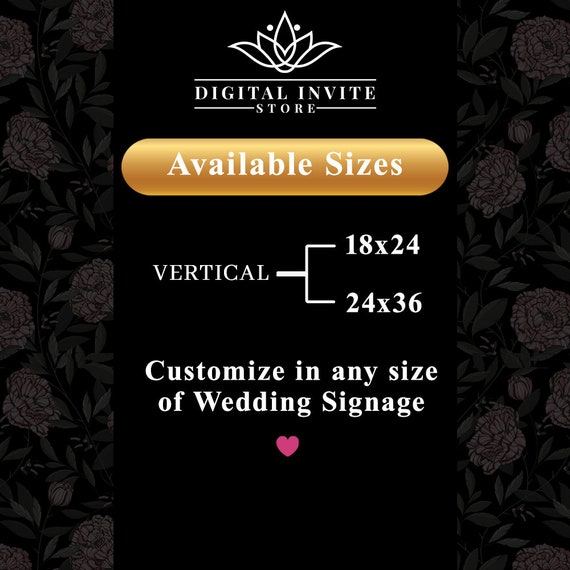The image is a section of a website that appears to be an advertisement for a digital invite store. The design features a black or dark gray background adorned with faint images of flowers and leaves, particularly noticeable on the right and left sides. At the top center, the store's logo is displayed, consisting of a symmetrical five-petal flower with two dots and the text "Digital Invite." Below the logo, "Store" is written in white lettering. Beneath this, a prominent yellow oval button with white text reads "Available Sizes." The advertisement then details size options vertically through a bracket connecting to the dimensions "18 by 24" and "24 by 36." Additionally, it offers customization for any size of wedding signage, all written in white text. The design is further accented by a small pink heart icon located towards the bottom of the graphic.